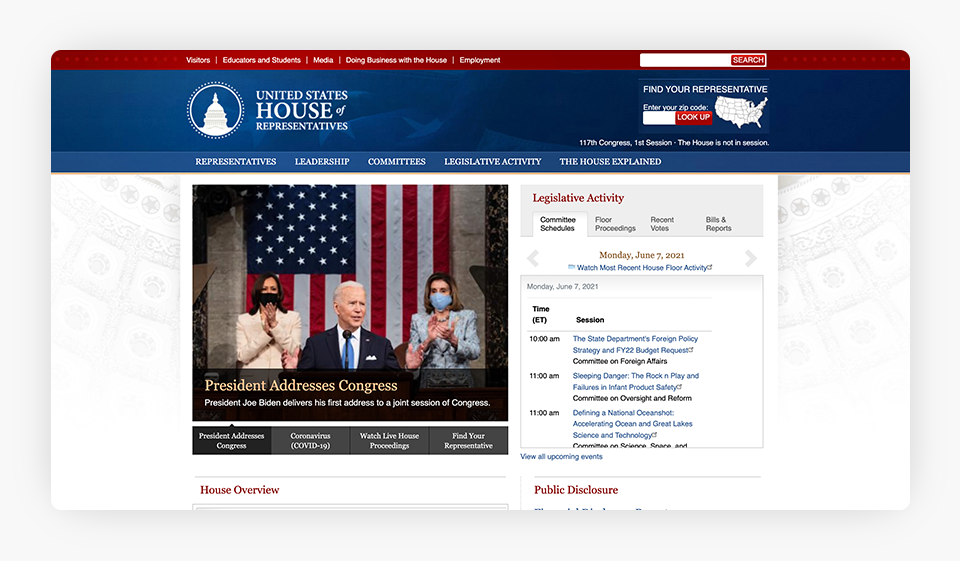The top section of the image features the header of a webpage with a red background. In the top left corner, there are white tabs labeled "Visitor," "Education and Student," "Media," "Doing Business with the House," and "Employment." On the top right, a red search button is accompanied by a white search box.

Below the header, the left side of the webpage has a blue background with the text "United States House of Representatives." On the right side of the header, instructions read "Find Your Representative and Type Your Zip Code," followed by a red button labeled "Look Up."

Underneath the header, the date "August 17th" is displayed, followed by the message "Congress In Session," then "The House is Not in Session." Below this, another set of tabs includes "Representatives," "Leadership," "Committees," "Legislative Activity," and "The House Explained."

On the left below these tabs is an image of President Joe Biden surrounded by clapping women. The background includes the American flag's colors of red, white, and blue. At the bottom of this image, yellow text reads "President Addresses Congress." Underneath, white text states, "President Joe Biden delivers his first address to a joint session of Congress."

Further down, there are additional tabs labeled "President Addresses Congress," "Coronavirus," "White House Proceedings," and "Find Your Representative." On the right side, there are sections for "Legislative Activity," "Committee Schedule," "Floor Proceedings," "Recent Videos," and "Bills and Reports."

At the bottom of the image, a date indicator reads "Monday, June 7th, 2021," followed by an invitation to "Watch Most Recent House Floor Activity: Session One." Schedule details are listed for various events in blue text, including:
- 10 a.m.: "The State Department Foreign Policy Strategy and FY22 Budget Request"
- 11 a.m.: "Sleeping Danger: The Rock 'n Play"
- 11 a.m.: "Advancing National Ocean and Great Lakes Science and Technology."

This structured layout presents an organized overview of the webpage dedicated to the United States House of Representatives.